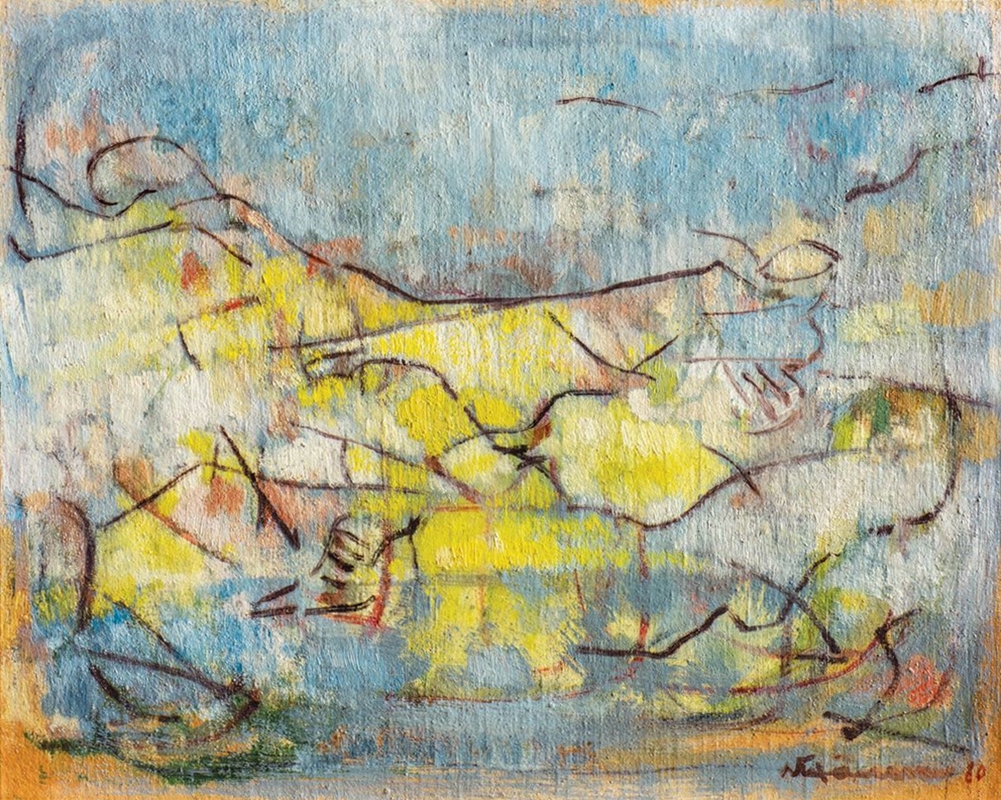This vibrant and abstract artwork, likely a hand-painted piece, prominently features a myriad of attractive colors forming an indistinct composition. Dominated by shades of blue at the top, transitioning to yellows in the middle, and culminating with a variety of colors including tan, orange, and patches of green towards the bottom left, the painting's colorful palette lends it an enigmatic allure. Although the exact imagery remains obscure and open to interpretation, some may perceive potential shapes such as individuals or birds against what could be a sky or layered rock formation. The piece lacks any text except for an artist's signature located at the bottom right. The overall abstract nature, combined with a harmonious blend of colors, particularly blue, yellow, white, orange, tan, green, and subtle gray tones, creates an engaging visual experience without any discernible objects.